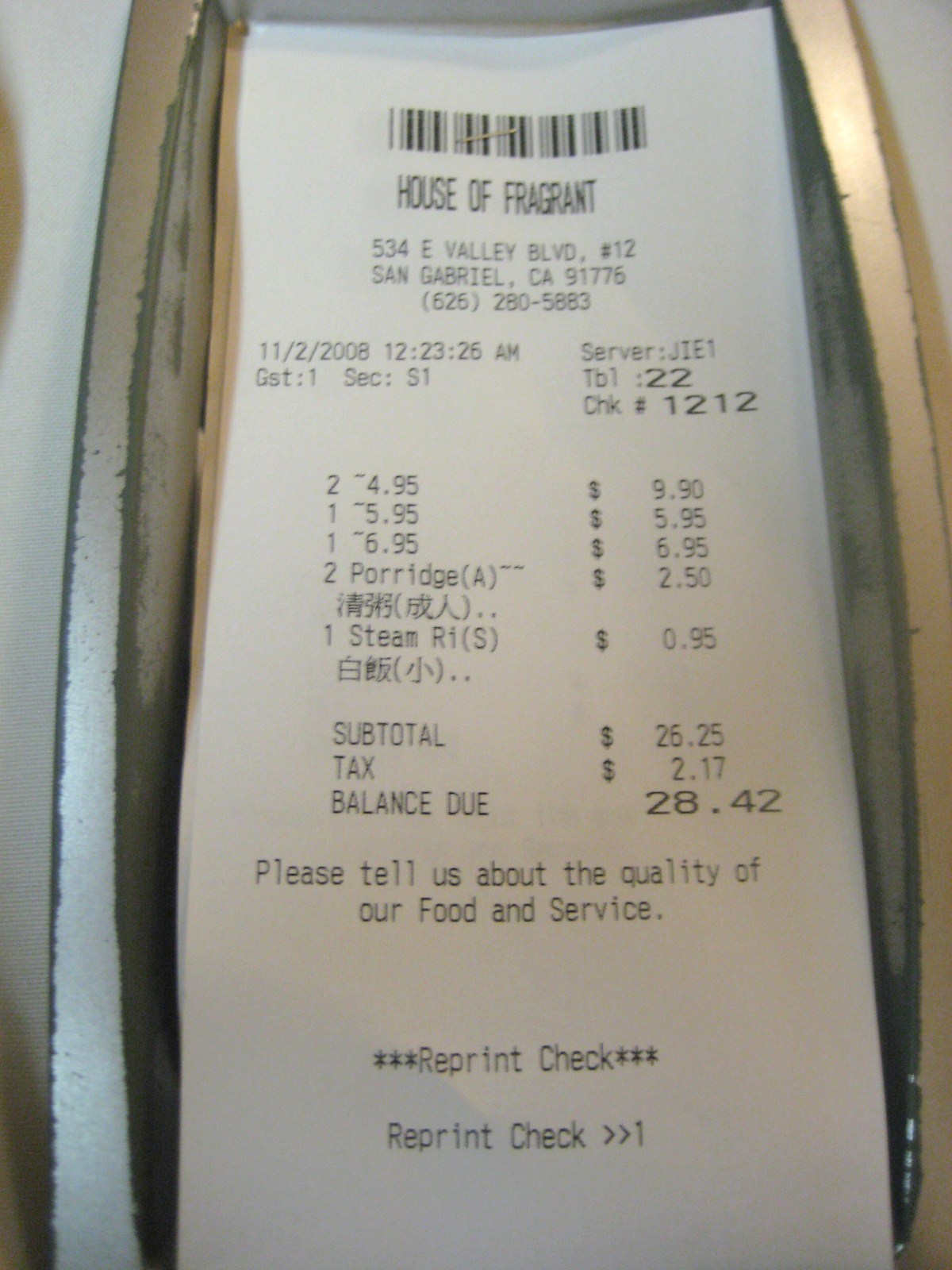This image showcases a white receipt placed inside a small cubby-like compartment, possibly within a vehicle, though the surroundings are cropped and not visible. The cubby features a gold-edged ridge creating a designated area for storing small items. The receipt itself is from "House of Fragrant," located at 534 East Valley Boulevard, Suite 12, San Gabriel, California, 91776, and bears the phone number 626-280-5883. The transaction occurred on November 2, 2008. Detailing a food order, the receipt includes specifics such as the server, table number, check number, and various itemized order details.